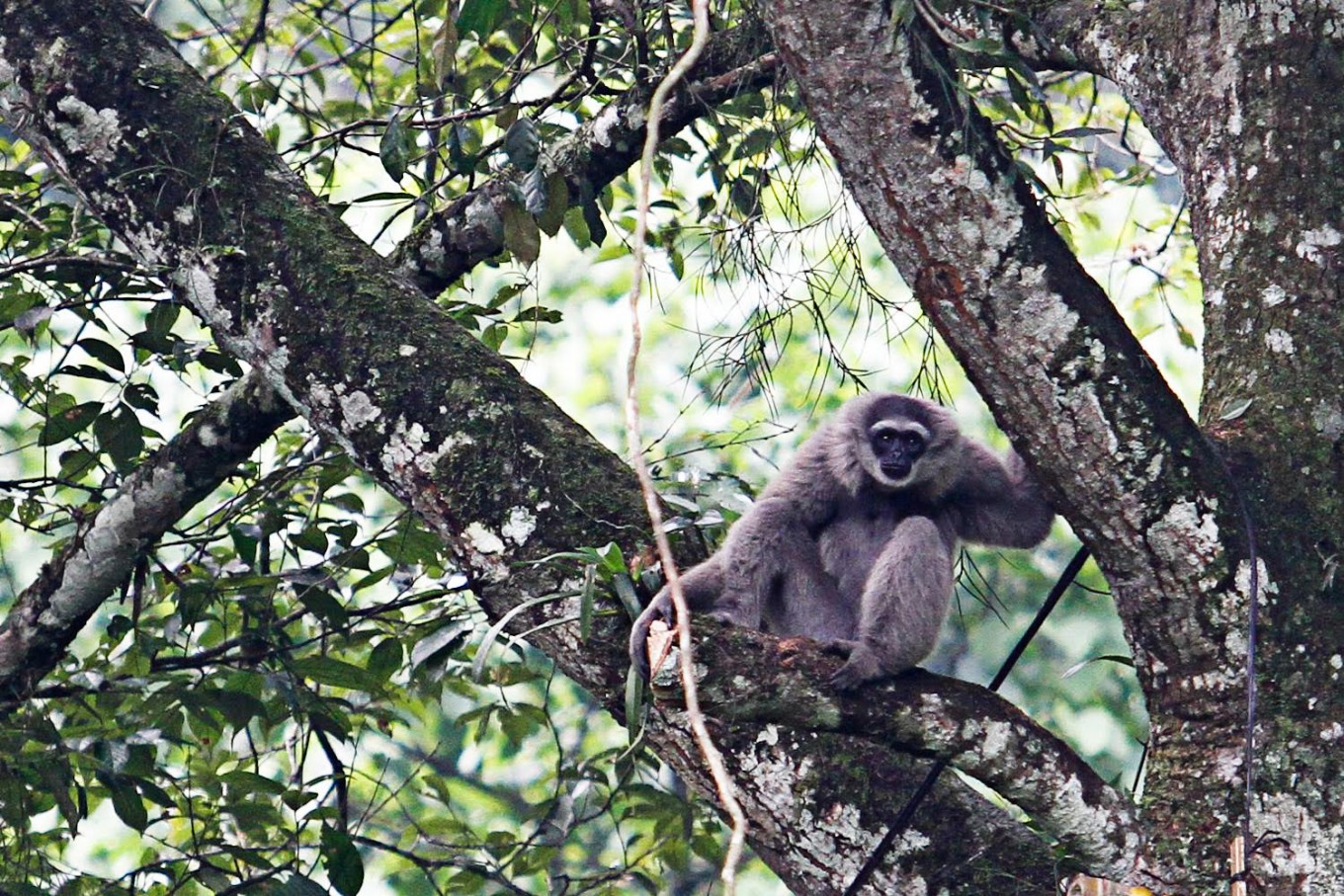In this close-up image, a small monkey with gray fur is perched in a large tree, gripping a thick branch with its right hand. The monkey's face is predominantly black with a distinctive white mask over its bushy eyebrows, and its black eyes stare directly into the camera. One of its black feet dangles over the branch. The scene is rich with detail, featuring moss of various colors growing on the tree's bark and a blurred light-colored branch or vine hanging in the background. The upper right of the photo is illuminated by sunlight, casting a natural glow over the out-of-focus trees and green leaves surrounding the monkey.